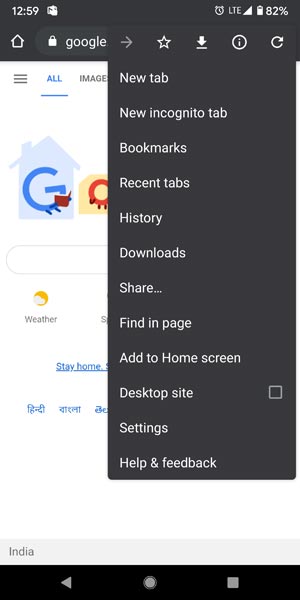This image is a detailed screenshot from a smartphone displaying a web browser's interface. The top header has a dark gray background. On the left side of the header, the time is displayed as "12:59." On the right side, there is a battery icon indicating an 82% charge level, alongside the LTE symbol representing an active wireless connection.

Beneath the header, there is a browser navigation bar on a dark gray background. On the left side of the navigation bar, an icon represents the home page. Next to this, in white font, the web page is identified as "Google." Also present in this bar, on the right side, is a drop-down menu icon, indicating additional options.

The main portion of the screenshot reveals an overlaid drop-down menu, an oblong rectangular shape stretching lengthwise across the screen. This menu displays various options in white font, listed from top to bottom:
- New tab
- New incognito tab
- Bookmarks
- Recent tabs
- History
- Downloads
- Share
- Find in page
- Add to home screen
- Desktop site
- Settings
- Help and feedback

Also visible in the background is the Google search engine homepage, partially obscured by the overlay of the drop-down menu. The visual elements cohesively represent a typical smartphone browsing experience.